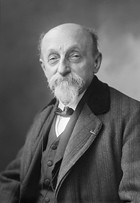This black and white photographic portrait captures an older man, posed diagonally with his left shoulder closer to the camera and his right shoulder further back. He is balding on top with some hair on the sides and back, complemented by a long white goatee and mustache. The man dons a three-piece suit, consisting of a white dress shirt, a vest with buttons in the middle, and an overcoat with a suit jacket underneath. He also wears a black bow tie or cravat. The background features a splotchy, photographic backdrop transitioning from gray to lighter, whitish hues. Notably, his face, marked with wrinkles and bags under the eyes, faces directly toward the camera, adding a sense of solemnity and character to the portrait, reminiscent of early 1900s attire and photographic style.